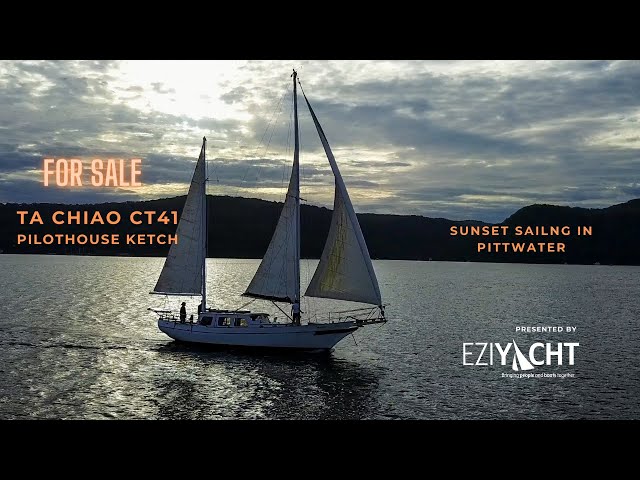The photograph captures an advertisement featuring a white yacht with three prominent sails—a large one in the middle, a smaller one at the front, and another at the back, cruising on a body of water. The scene is set during the day, though the sun is obscured by clouds, casting a darker, overcast light on the landscape. In the background, there are dark, mountainous areas, accentuating the yacht's presence in the foreground. 

To the left side of the image, "For Sale" is displayed in yellow text, overlaid like a watermark against the sky, followed by "Ta Chiao CT41" in orange text and "Pilot House Ketch." On the right side, against the backdrop of a mountain, is the text "Sunset Sailing in Pittwater." Below this, in white text, is "Presented by EZIY," where the 'A' in 'EZIY' is stylized to resemble a yacht sail, and beneath that, there is text that reads "C-H-T" along with the phrase "Bringing People Something Beach," though the complete phrase is unclear.

The yacht itself shows two individuals—one standing on the left side near one of the sails and another person near the mast. The deck features a pilot house and various outriggings, adding to the vessel's detailed structure. The overall ambience suggests a sophisticated and serene sailing experience being offered for sale.